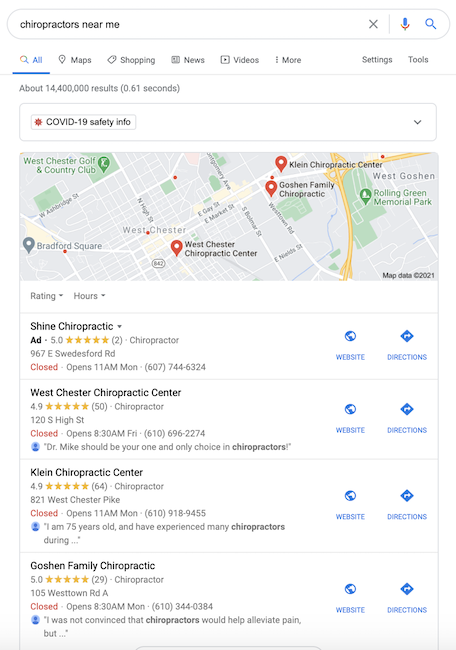A screenshot of a Google search results page for "chiropractor near me." At the top, multiple tabs are visible including All, Maps, Shopping, News, Videos, More, Settings, and Tools. The page displays approximately 14,400,000 results in 0.61 seconds. There is a rectangular box prominently featuring COVID-19 safety information with a small red dot to the left and a dropdown arrow to the right.

Below the safety information, a map is displayed with markers indicating various chiropractic centers in the area. The bottom right corner of the map shows “Map data ©2021.”

Highlighted locations include:

1. West Chester Chiropractic Center
2. Goshen Family Chiropractic
3. Klein Chiropractic Center
4. West Goshen
5. Rolling Green Memorial Park

Additionally, a street view is partially visible. 

A rating and hours of operation are displayed for Shine Chiropractic, showing 5.0 stars based on 4 reviews. The address is 927 East Westford Road, and it is marked as closed with reopening at 11 a.m. on Monday. 

West Chester Chiropractic Center is mentioned again with a rating of 4.9 stars based on 50 reviews. Klein Chiropractic Center follows with a rating of 4.9 stars and 64 reviews. Lastly, Goshen Family Chiropractic boasts a 5-star rating from 29 reviews at 905 West Town Road. 

A personal note at the bottom of the search results reflects skepticism about the efficacy of chiropractic treatment for pain relief.